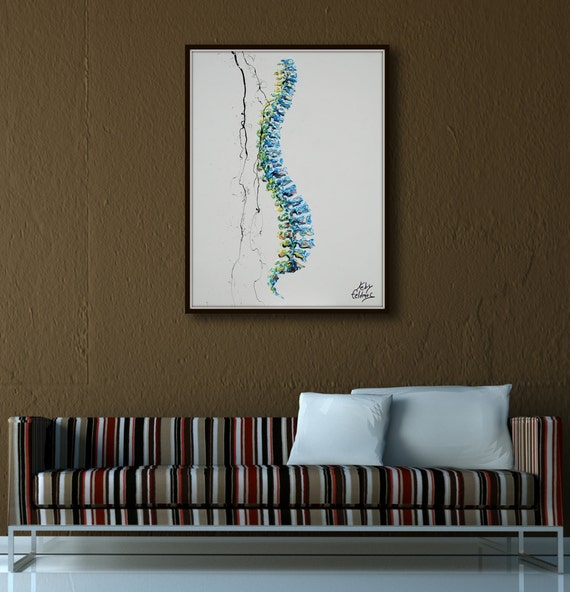The image features a modern sitting area with a long, vertically striped couch spanning the full width of the frame. The couch's stripes include colors such as white, black, tan, red, and beige, and it rests on a sleek metal frame with square silver metal legs. Positioned on a shiny white marble floor, the couch has two white pillows on its right side: one square throw pillow and one long rectangular pillow.

Behind the couch is a dark brown textured wall, which serves as a backdrop for a framed piece of art. The painting, set within a thin black frame, features a white background and depicts what appears to be the human spine, artistically rendered in blue with green and yellow highlights. The spine is curved, adding a dynamic visual interest to the piece. The painting is signed in the lower right corner, although the signature is illegible. The overall scene creates a stylish and contemporary aesthetic, suitable for either a living room or a modern office setting.